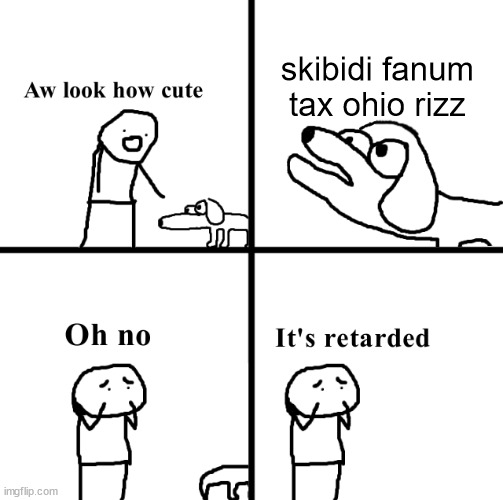In this black-and-white illustration, a large plus sign divides the image into four distinct quadrants. Each section contains a unique scene, all created with black outlines on a white background. 

- **Top Left Quadrant:** Features the caption "Aww, look how cute," accompanied by a simple drawing of a figure with a square body and a round head, reminiscent of a stickman, complemented by a small weenie dog beside him.

- **Top Right Quadrant:** Showcases the dog speaking peculiar phrases: "Skibbadee," "Phantom," "Tax," "Ohio," and "Riz."

- **Bottom Left Quadrant:** Depicts the square-bodied figure with hands on his face, expressing dismay with the caption "Oh no," as the weenie dog turns away and starts to walk off.

- **Bottom Right Quadrant:** Focuses solely on the distressed figure with hands on his face, lamenting the situation with the caption "It's retarded."

The minimalistic art style employs black outlines for all drawings, leaving the interiors of the characters unfilled, creating a stark, contrasting visual narrative.